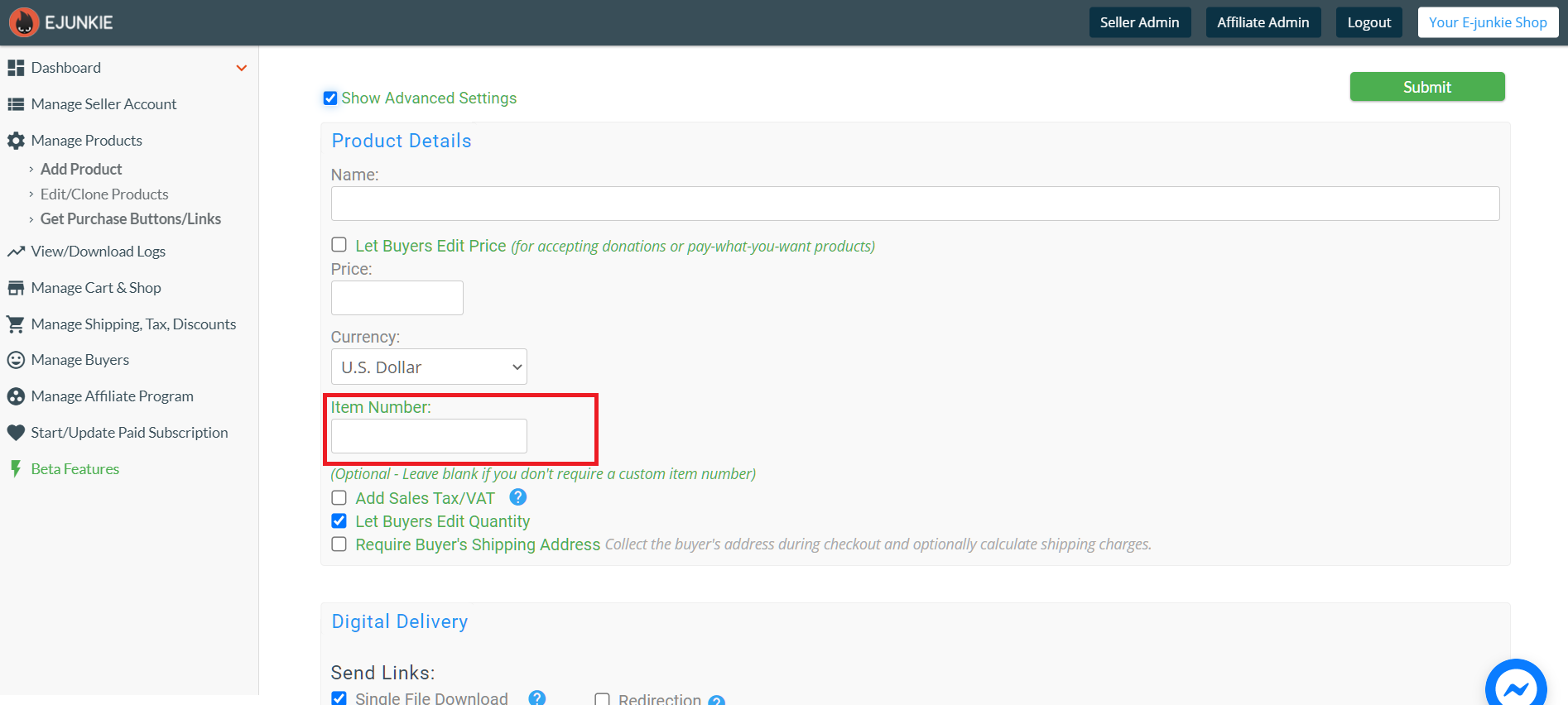The webpage screenshot showcases the eJunkie platform, prominently displaying the eJunkie logo at the top left corner—a circular orange background featuring a stylized, black smiley face with eyes that appear to be glaring. The navigation bar includes options for "Seller Admin," "Affiliate Admin," "Logout," and "Your eJunk Shop."

Below the navigation bar, the dashboard area is highlighted with an orange drop-down button. Additionally, there are several functional buttons available, including "Manage Seller Account," "Manage Products," "Add a Product," "Edit or Clone a Product," and "Get Purchase Buttons/Links." Users can also "View/Download Logs," "Manage Cart and Shop," "Manage Shipping, Tax, and Discounts," "Manage Buyers," "Manage Affiliate Program," "Start/Update Paid Subscription," and access "Beta Features" identified by a green icon.

The main focus of the page is the "Product Details" section. Here, users can input the product's name, price, currency, and item number—the latter outlined with a red box, signaling its importance. There are additional options such as "Add Sales Tax," "Let Buyers Edit Quantity" (which is checked with a blue checkmark), and "Require Buyer's Shipping Address," which includes details about collecting the buyer's address during checkout and optionally calculating shipping charges. Another notable feature is the "Digital Delivery" option, which allows sellers to send links for single file downloads or redirect buyers.